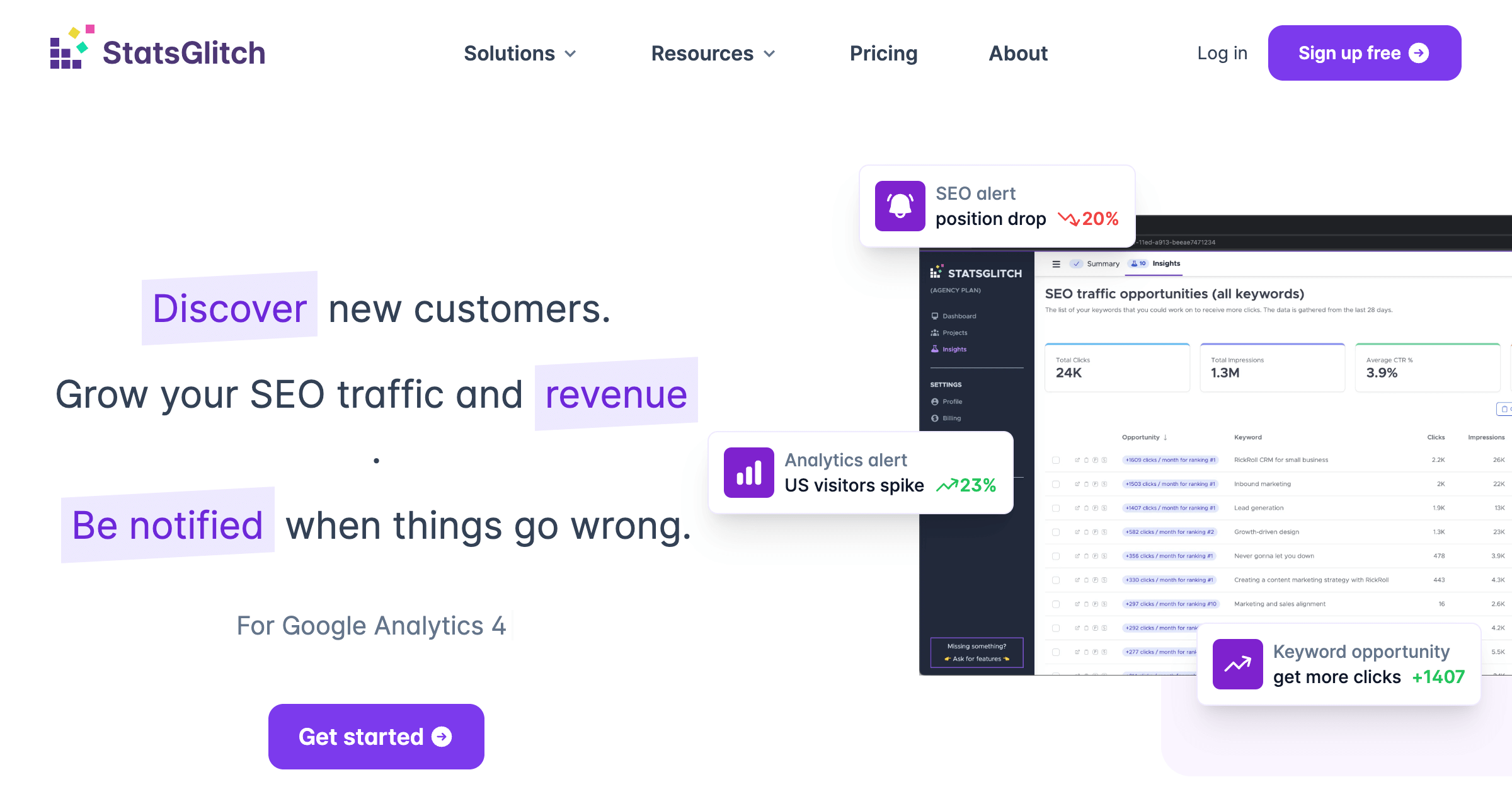The image captures the homepage of a website called Stats Glitch. In the top left corner, the logo and brand name are prominently displayed. To the right of the logo are dropdown menus labeled "Solutions" and "Resources." Further right, additional menu items include options for "Pricing," "About," and "Login," with a purple "Sign Up for Free" button at the far right. 

Beneath this navigation bar on the left-hand side, impactful introductory text reads: "Discover new customers, grow your SEO traffic and revenue, be notified when things go wrong." The words "discover," "revenue," and "be notified" are highlighted in purple for emphasis. Below this, there is mention of Google Analytics 4, accompanied by another purple "Get Started" button.

To the right of this text block, there is a miniature window featuring a gray banner on its side and a white central area. Surrounding this window are notification pop-ups that signify various alerts:
- A bell icon alert indicating an SEO position drop of 20%.
- A chart icon alert showing a 23% spike in US visitors.
- A "keyword opportunity" notification suggesting actions to get more clicks.

The design effectively uses accents of purple and clear, informative visuals to engage users and guide them through the offerings of Stats Glitch.